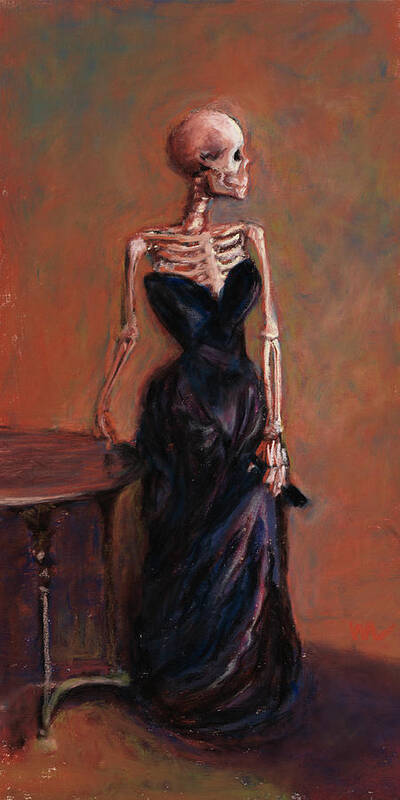The image showcases a detailed and evocative painting of a female skeleton adorned in a sleeveless, black velvet dress with a V-neck that drapes over the ribcage. The skeleton stands in an elegant, almost parodic imitation of a famous artwork, possibly Whistler's. With its head turned to the right, the skeleton's left hand delicately holds part of the dress, while the right arm gracefully leans on a round, brown wooden table with four legs. The background of the painting is a rich mix of beige, brown, red, and blue hues, adding depth and contrast to the scene. The floor beneath the skeleton is subtly suggested, completing the composition's ambiance.